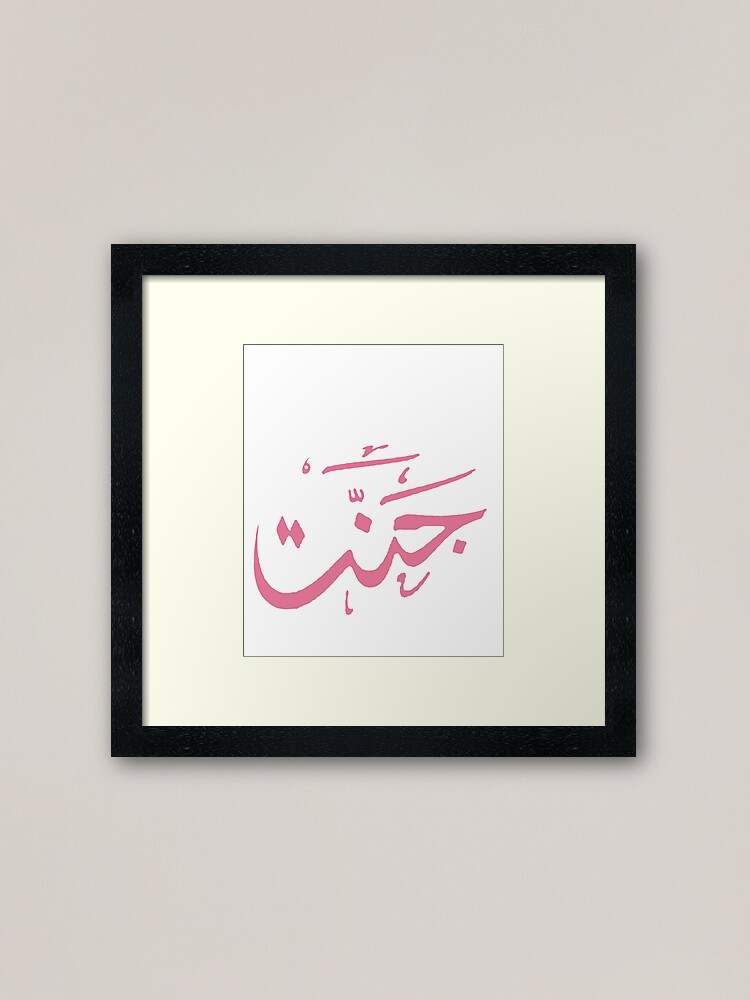The image displays a black-framed picture hanging on a tan wall. The frame encases a cream-colored matting that surrounds a white rectangular section hosting intricate, pinkish-red markings, possibly of Asian or Arabic origin. These markings include squiggly lines, diamonds, and what appears to be a 'W' shape, among other patterns. The symbols and lines dominate the white background, organized with two diamonds on the left and one in the center, and various squiggles and shapes distributed throughout. Notably, there is a prominent thick, swirling line with an arrow towards the bottom. Despite the detailed patterns, the image provides no translation, leaving the exact meaning of the symbols unknown to the observer. The painting is well-centered within the frame, leading to a minimalist yet enigmatic design.